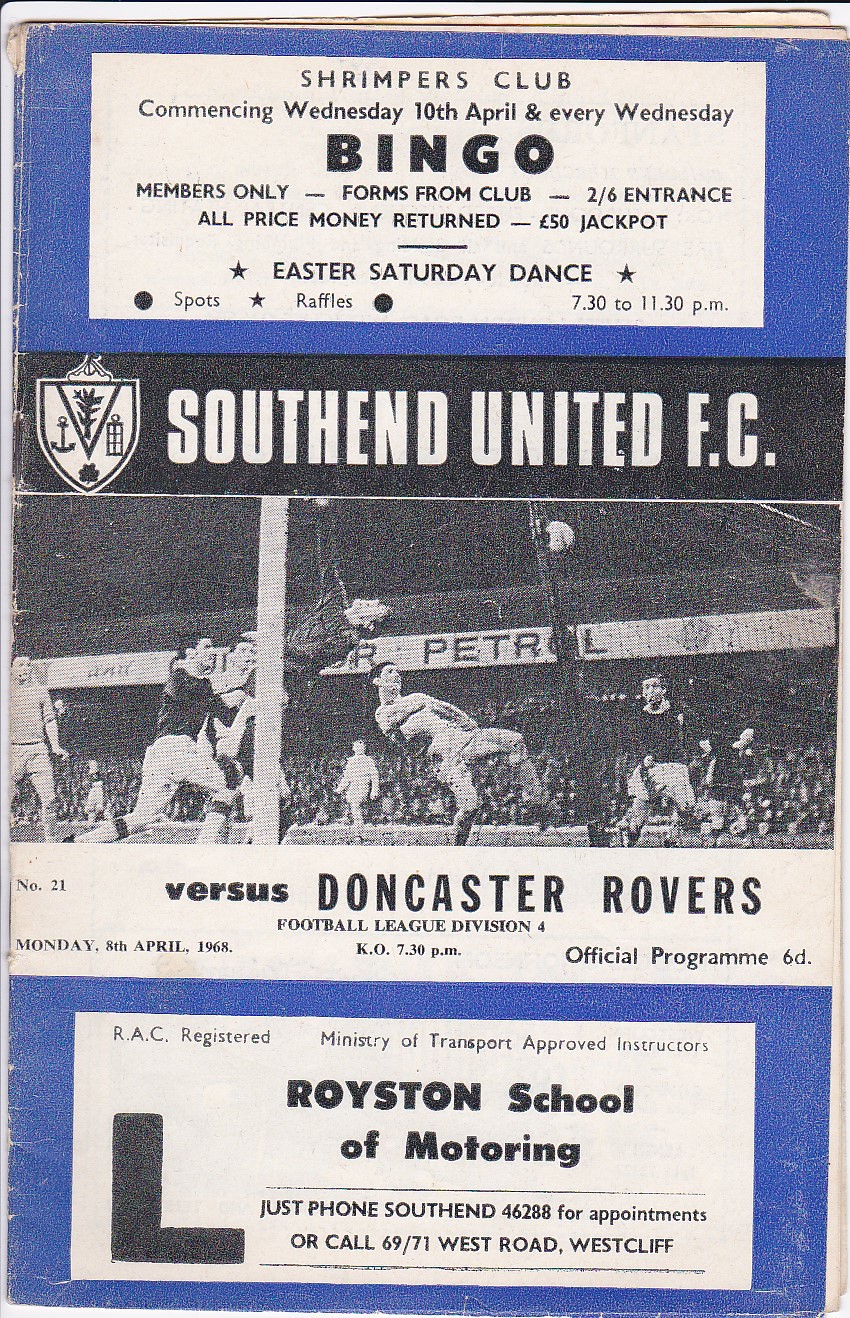This image is a scan of an old program cover, largely in black and white with prominent blue sections at the top and bottom. The top blue section features a white box with black lettering, announcing the "Shrimper's Club," commencing Wednesday, 10th April, and continuing every Wednesday, with a bold "BINGO" for members only. It details various club-related activities, including forms from the club, entry fee specifics, a 50-pound jackpot, and an Easter Saturday dance from 7:30 to 11:30 PM.

Centered on the program, a black-and-white photograph captures a dynamic soccer game, showing several players actively engaged in play, with a crowd visible in the background. Above the image, "Southend United FC" is displayed in white letters on a black background. Below the photograph, more text specifies that Southend United FC is set to face Doncaster Rovers in a Football League Division IV match on Monday, 8th April 1968, at 7:30 PM. Additionally, the cover indicates it is the "Official Program" priced at 6D.

The bottom blue section contains advertisements, including one for the Royston School of Motoring, described as "RAC Registered Ministry of Transport Approved Instructors." It provides contact details, urging readers to phone Southend at 46288 for appointments or visit 69-71 West Road, Westcliff.